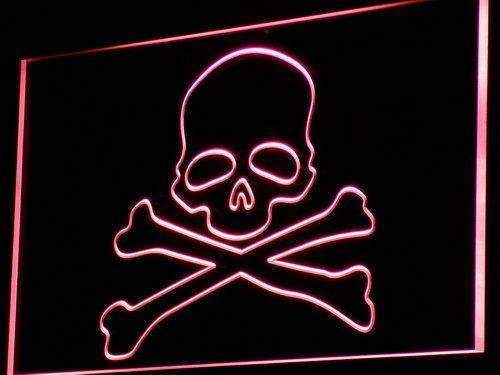The image depicts a neon sign with a skull and crossbones design, set against a solid black background. The focal point is a light pink, angled rectangle containing the outline of a skull. The skull includes defined eye sockets, a nose frame, and a mouth area, drawn in light pink LED. Directly below the skull, two femur bones cross each other, completing the classic crossbones motif. The entire pink outline gives the impression of a flag, adding a unique touch to this simplistic yet striking visual.